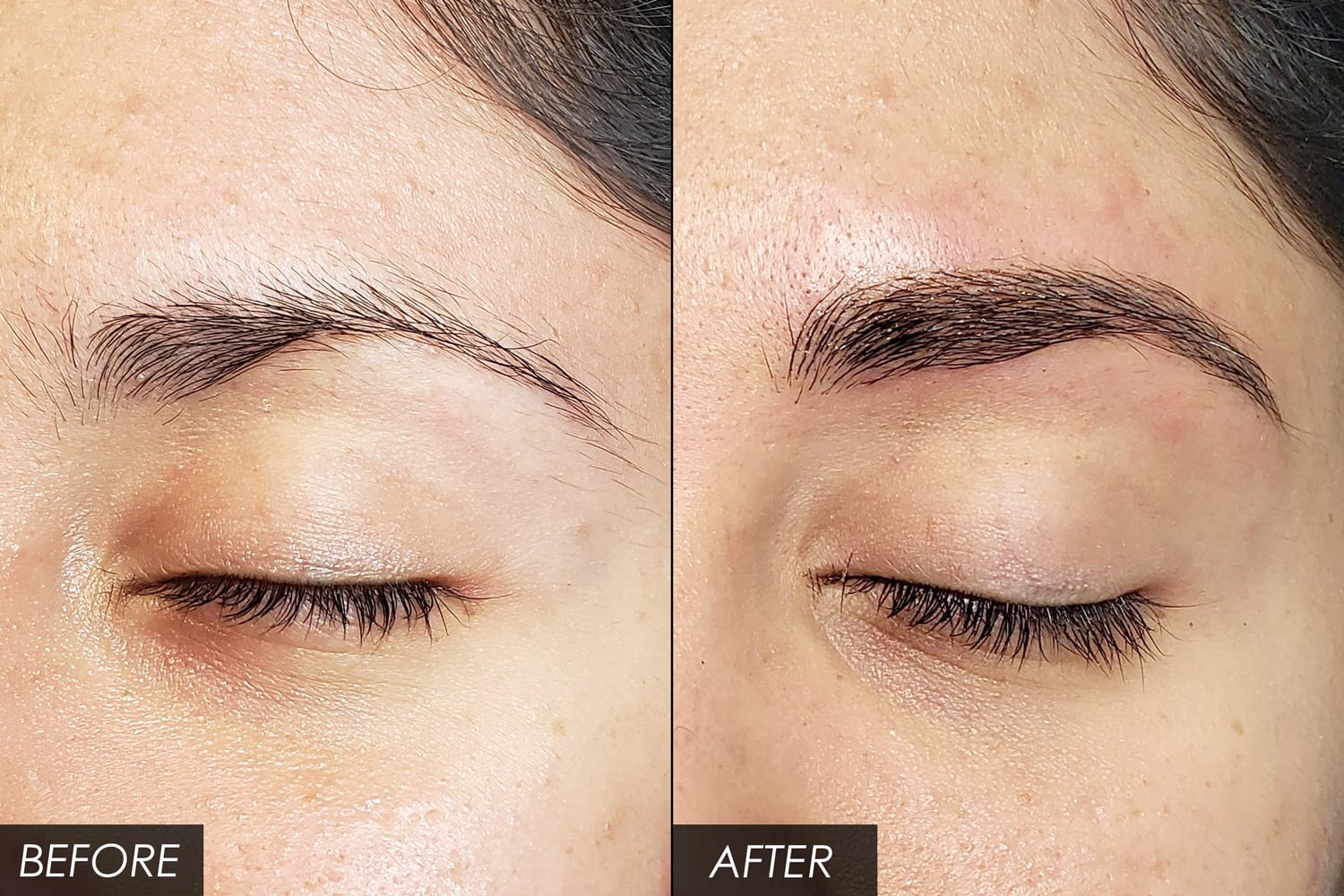This image is a before-and-after comparison capturing a woman's eyebrow transformation, likely due to a microblading procedure. In the 'before' image, located on the left, the woman's eyebrow appears very thin and spotty, with her eyelid closed, showcasing long eyelashes and even-toned skin. Her brown hair frames the sparsely populated eyebrow. In the 'after' image on the right, the eyebrow is significantly fuller and darker, with a beautifully defined shape. The skin around the eyebrow appears slightly red and puffy, indicating a recent procedure. Despite the redness, her eyelashes remain impressive, and the improved eyebrow adds to her overall refined look. The only text on the image is a black box with white letters reading "before and after," positioned to emphasize the eyebrow enhancement. This close-up of the top right-hand section of her face effectively showcases the dramatic improvement, making it a compelling visual likely used to highlight the success of a microblading business.